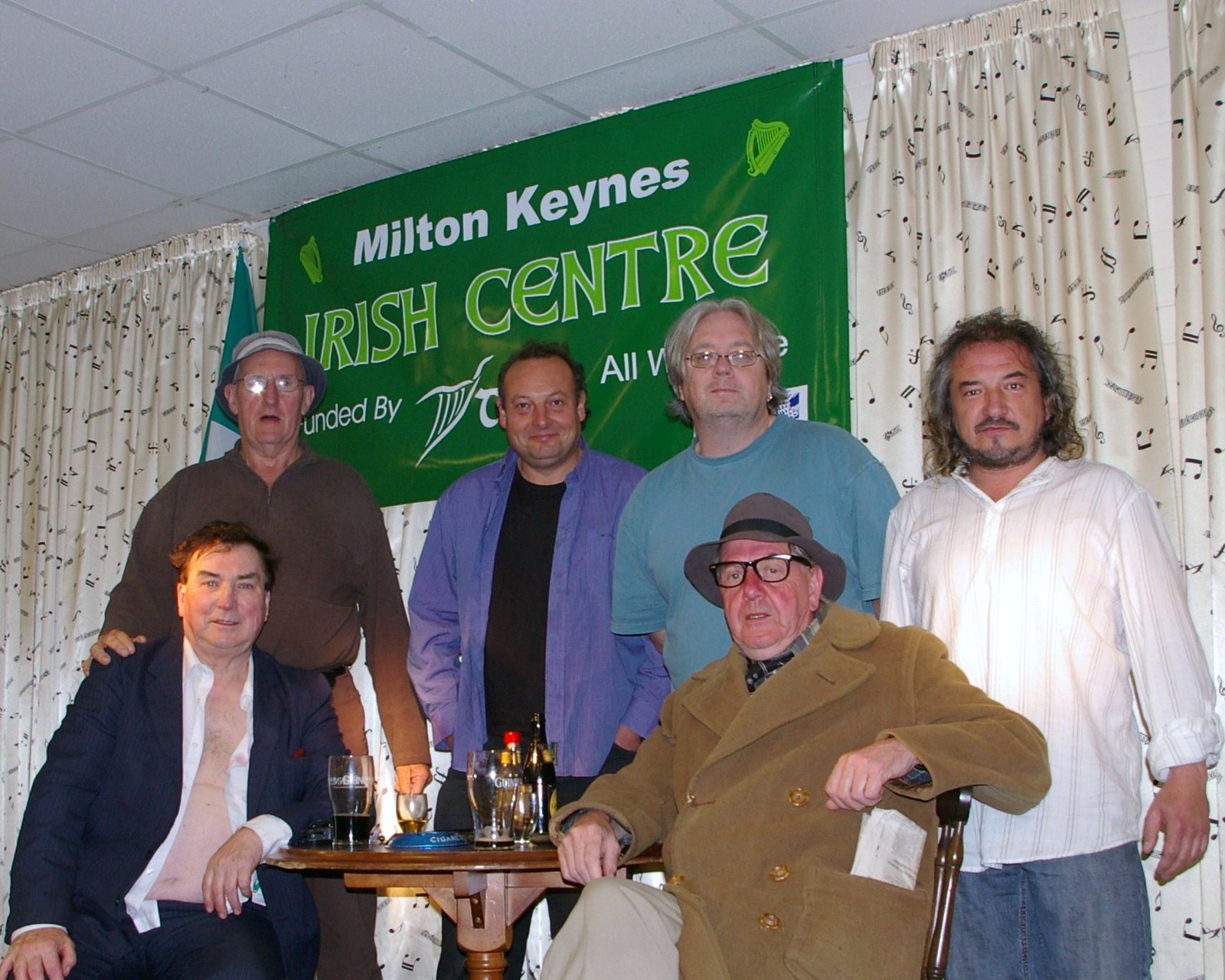In this clear and brightly lit image, a group of six men are posed around a small wooden table adorned with bottles and glasses of beer. The setting appears lively with natural light contributing to its brightness. In the background, a draped curtain with music notes frames a green banner that reads "Milton Keynes Irish Centre" in white and green text. Four men are standing while two are seated, all looking towards the camera. Standing from left to right: a man with a light gray hat, glasses reflecting light, and a brown jumper; a man next to him with black hair, wearing an unbuttoned blue shirt over a black t-shirt and smiling; another man with longer gray hair and glasses in a light teal shirt; and on the far right, a man with long black and gray hair, a beard, wearing a white striped shirt and blue jeans. Seated at the front left is a man with brown hair, his white shirt open at the chest beneath a blue jacket, smiling, with one arm resting on the table. To his right, another seated man wearing a gray cap, black glasses, a heavy brown coat, and khaki pants, is looking towards the camera. The background complements the convivial scene with a banner signifying the location, adding context to the gathering.